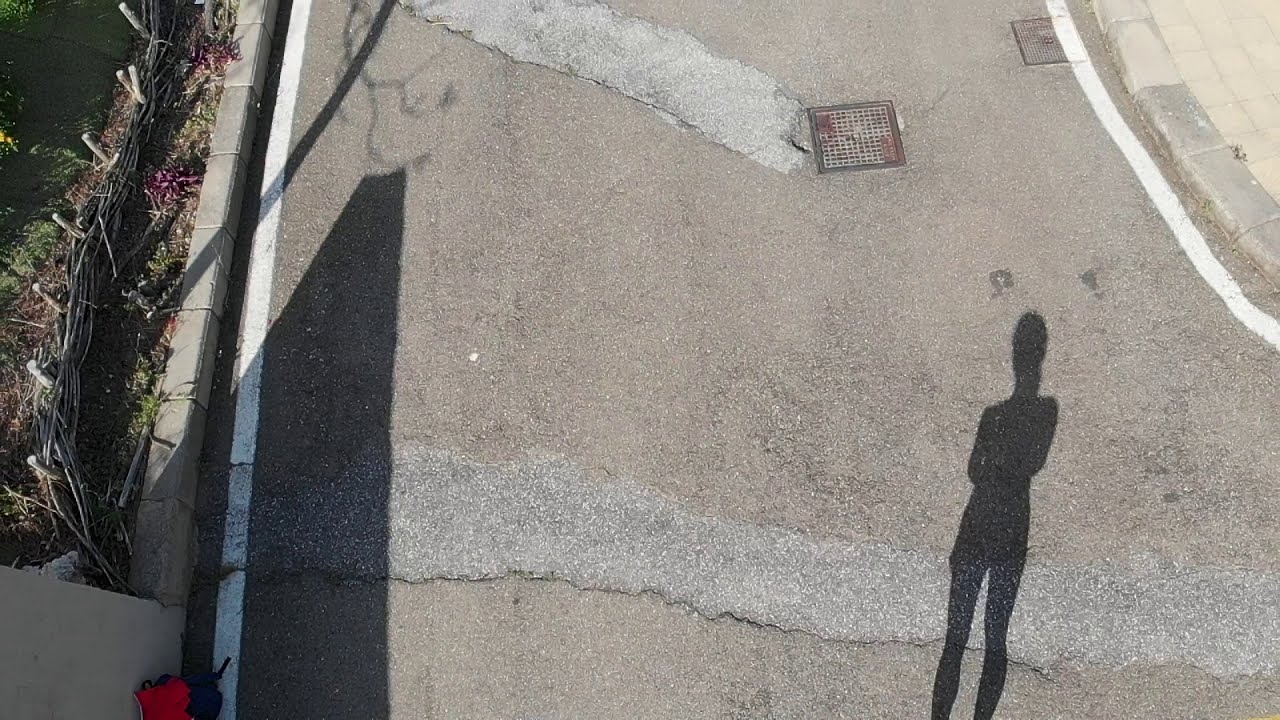This aerial image showcases a light gray, paved road running vertically through the center. The road surface is marked with numerous cracks and a slightly darker color adjacent to them. Each side of the road features white painted stripes. On the top right, there is a section of tan square-tiled sidewalk adjacent to the road, and a light gray metal grate is also visible. The left side of the road is bordered by a grassy area, enclosed by rectangular bricks, and accompanied by some garden plants near a small wooden picket fence. In the bottom left of the image, there is a red and blue backpack sitting near a concrete slab. Additionally, on the right side towards the bottom corner, a dark shadow of a thin woman is clearly visible cast on the road, adding a dramatic effect to the scene.